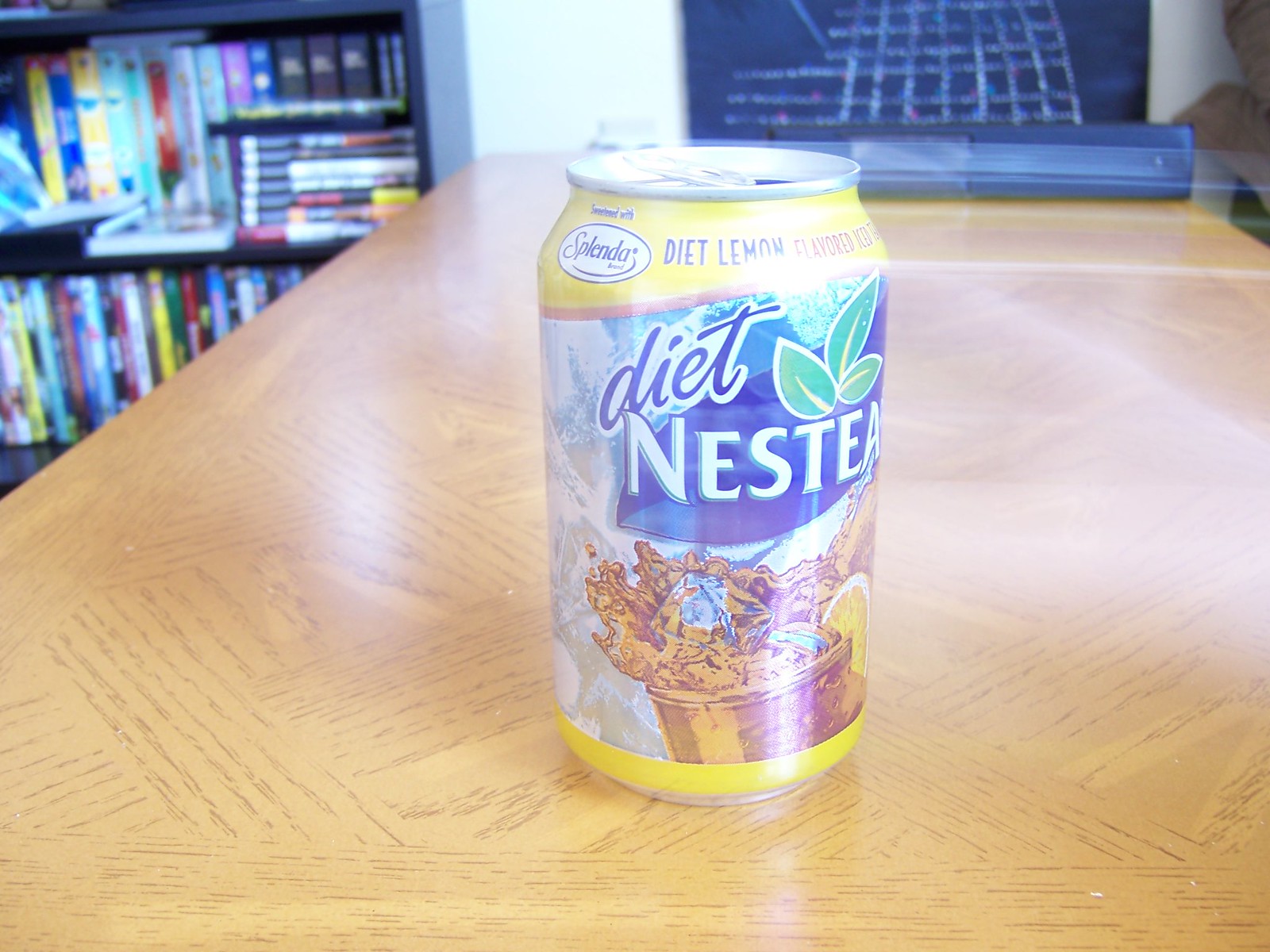A close-up image features a vibrant can of tea resting on a brown and golden tabletop. The can is predominantly designed in shades of yellow and blue, offering a visually appealing contrast. Prominently displayed on the front of the can is an enticing illustration of a cup filled with iced tea, complete with two ice cubes and a wedge of lemon, capturing the refreshing essence of the beverage. The text on the front of the can reads "Dietness Tea," accented by three green leaves that rest delicately atop the word "mess Tea." Additionally, the yellow portion at the top of the can clearly states "Diet Lemon Flavored Tea," informing consumers of the beverage’s flavor.